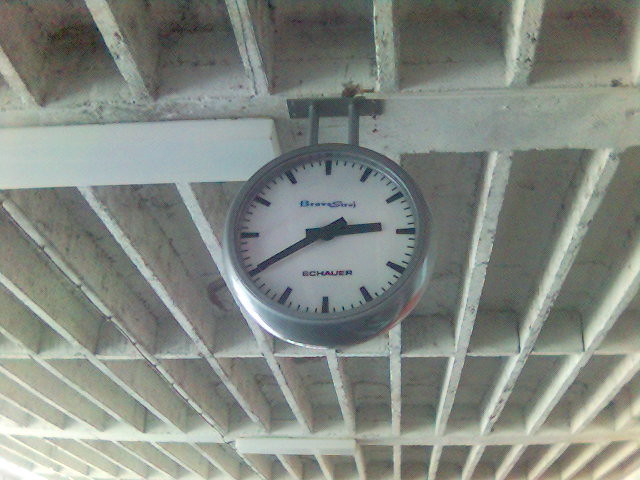The image depicts a rugged, off-white ceiling composed of exposed beams and rafters, with the paint chipping off to reveal the underlying wood. The ceiling has several rows of beams, intersected by cross-boards, giving it a textured and patterned appearance. Hanging from one of these beams is a gray metal clock. This analog clock features a circular body, a white face with large black hash marks denoting the hours and smaller ones denoting the minutes. The hour and minute hands are black, currently pointing to around 2:40. The clock has the word "E-C-H-A-U-E-R" above the number six position. The overall scene gives a sense of rustic charm mixed with functional simplicity.